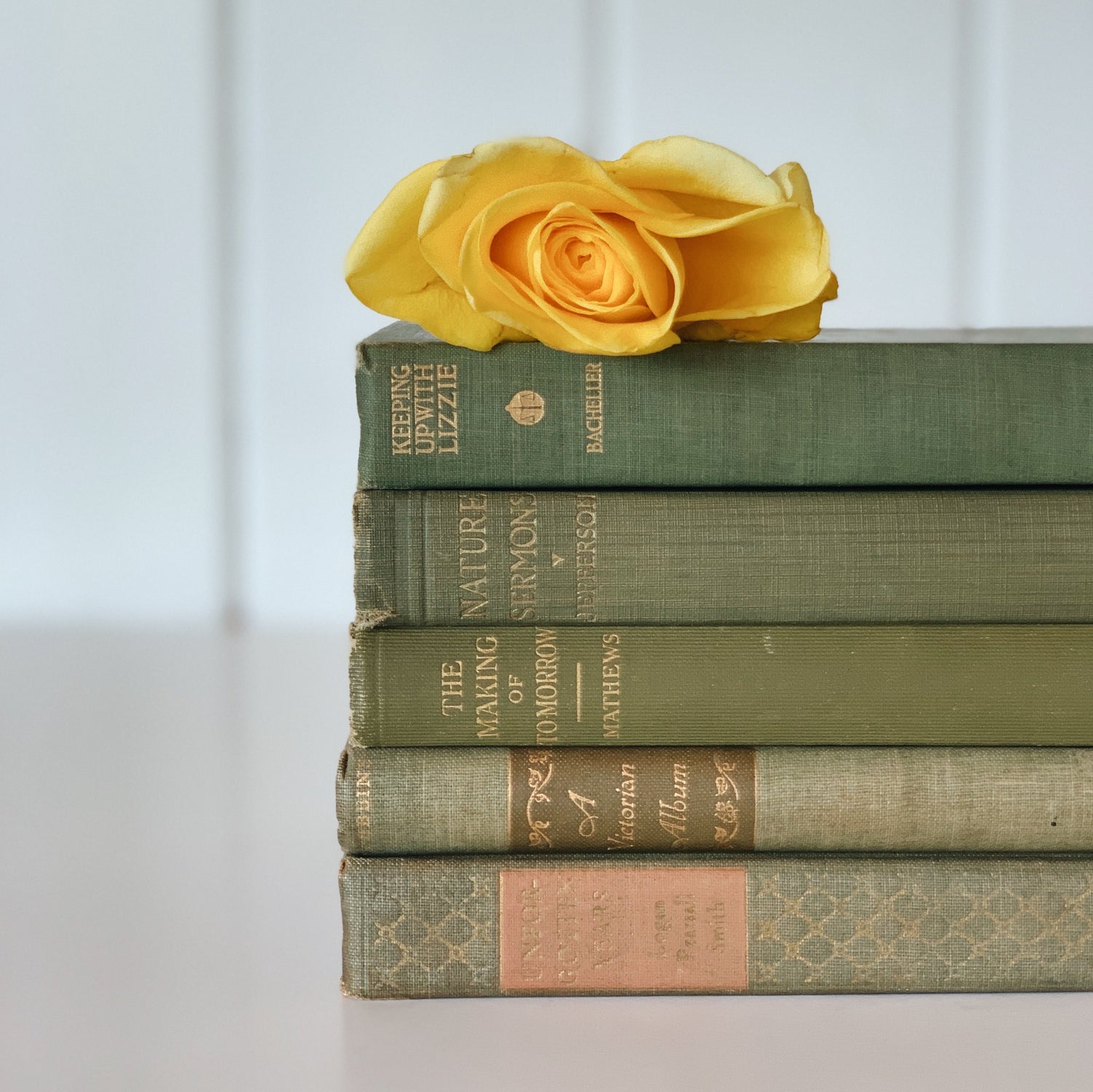In this color photograph, five hardcover books, worn and aged, rest on their sides atop a light gray table, against a sparse white wall. Each book, mostly clad in green with some pinkish tints, shows signs of wear across their top edges. From the bottom up, the visible titles are "A Victorian Album," "The Making of Tomorrow" by Matthews, "Nature's Sermons," and "Keeping Up With Lizzie." The title of the bottom book is unclear due to the worn lettering. Crowning this stack of books is a slightly wilted yellow rose, with no stem visible. The stark background and surface emphasize the vintage charm of the books and the delicate beauty of the rose, which appears almost symbolic amid the serene setting. There are no people or animals present in the image.